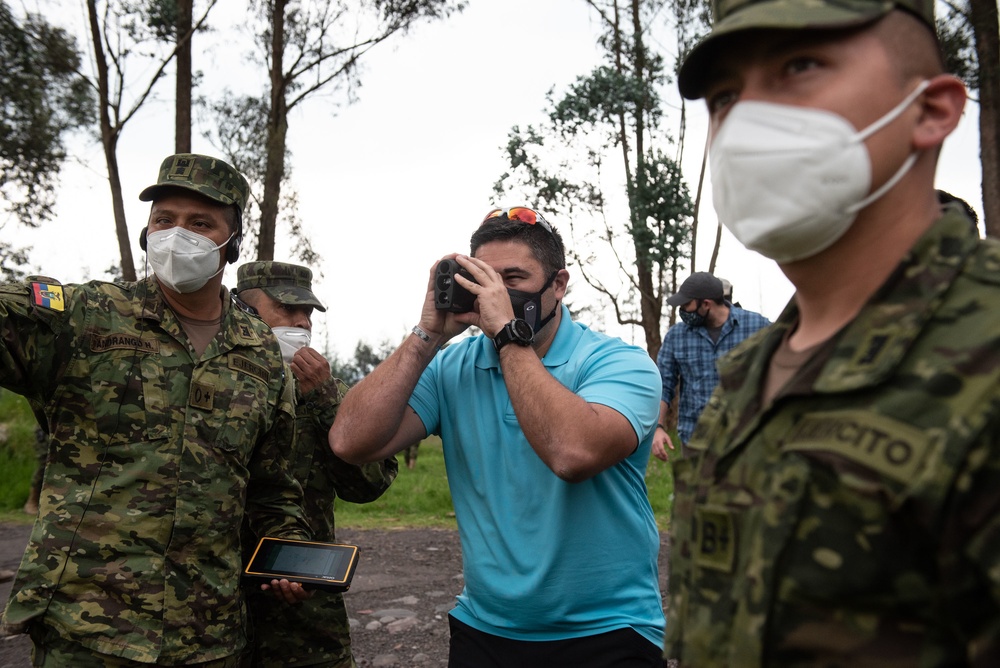The image is a horizontally aligned rectangular photograph depicting a group of men standing on a gravel surface. At the forefront, three men are wearing camouflage military uniforms with white masks covering their noses and mouths. One of these soldiers, positioned on the left, is pointing ahead and holding a yellow, blue, and red badge on his arm. He is clutching a large digital rectangular device, possibly a GPS, in his left hand. In the middle of the group is a man of Latino descent, who stands out due to his attire. He is dressed in a light blue short-sleeved polo shirt and brown pants or shorts, with a black fabric mask and orange-tinted sunglasses perched on his forehead. This man is taking a picture or filming through a digital camera or binoculars. Behind him, another man dressed in a blue plaid shirt and gray baseball cap is visible, also wearing a black mask. On the right side of the image, close-up of another soldier's chest displays a blurry name, "Sedo," on his camouflage gear, with a brown t-shirt peeking out from underneath. All the men are focused intently to the left, observing something out of the frame.